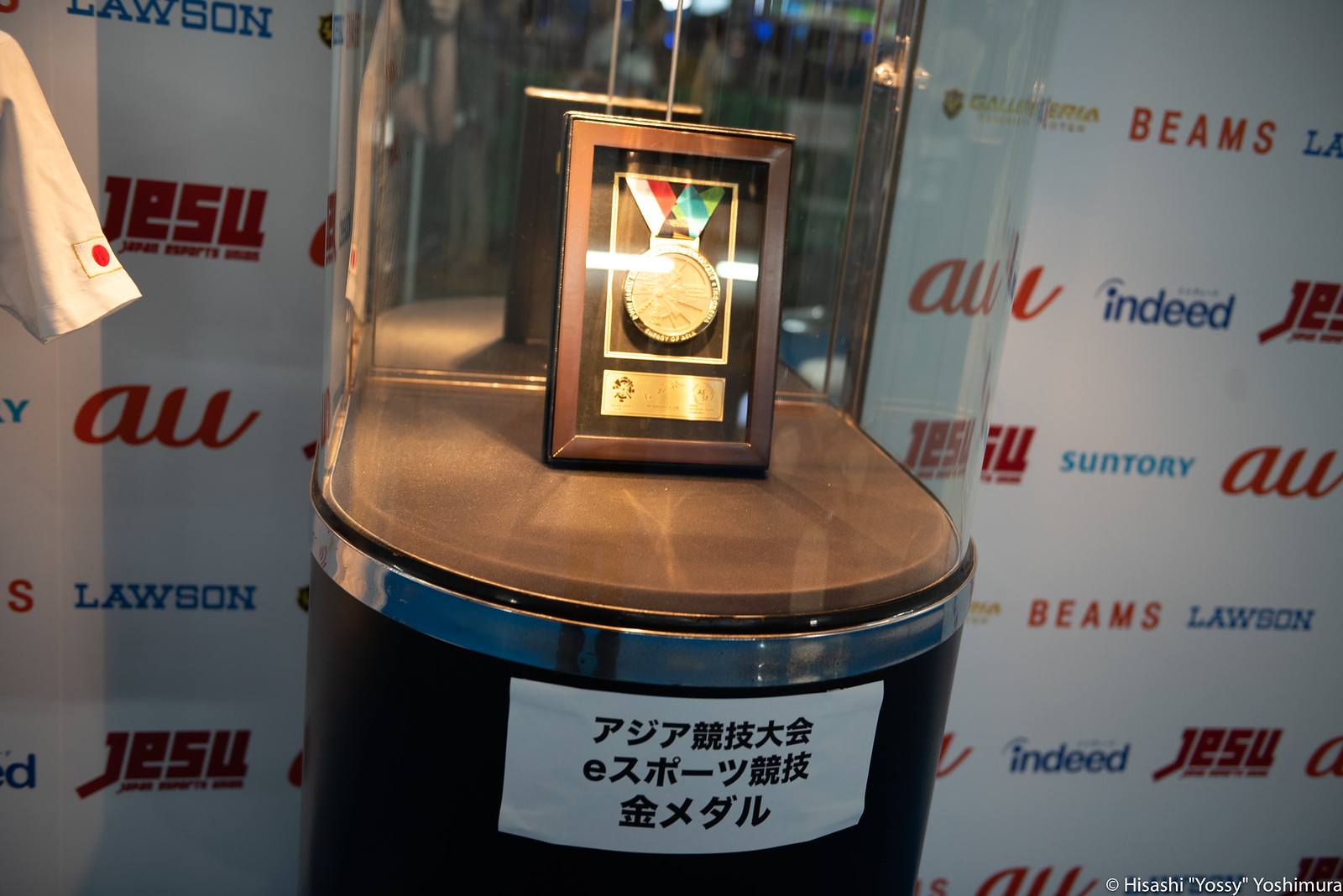The image showcases a detailed display case set against a white banner filled with sponsor logos including Beams, Indeed, Suntory, Lawson, and Jeju. The logos are presented in red and blue text on the banner. The display case itself is constructed from a combination of brown wood and glass. On the wooden base of the case, there's a white label with black Chinese characters identifying the content above. Enclosed within a curved glass top, the focal point of the display is a gold medal framed in wood, with ribbons in white, red, and green descending diagonally from the medal. The case is designed to appear like a typical plaque display, and the gold strip beneath the medal further signifies the achievement it represents. This carefully enclosed medallion presentation is both protective and elegant, making it the centerpiece against the backdrop of prominent sponsor names.